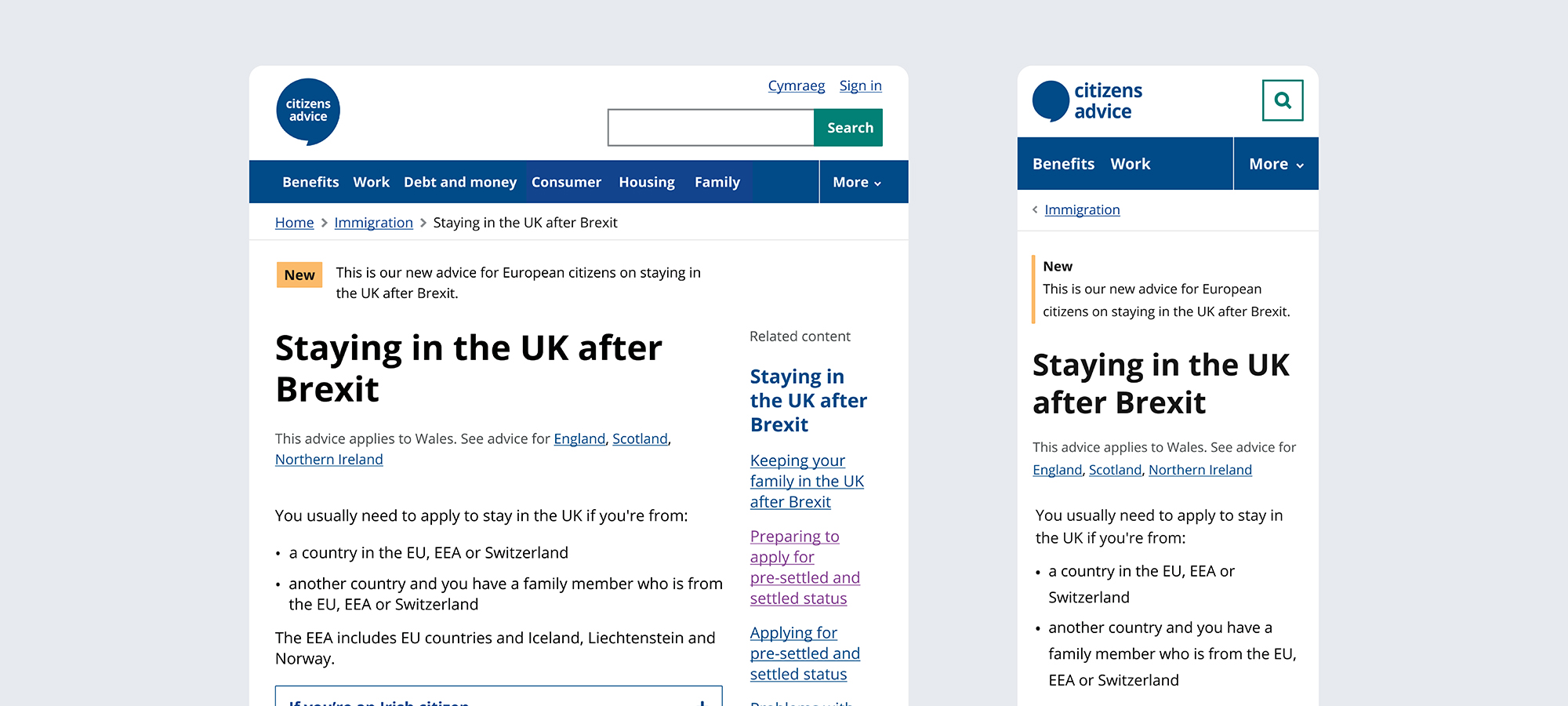Here's the cleaned-up and detailed caption:

"This image is from Citizens Advice, displaying their web page focused on providing guidance for European citizens on staying in the UK post-Brexit. The layout features a sign-in option and a search bar with a green search icon. The main navigation menu includes categories such as Benefits, Work, Debt and Money, Consumer, Housing, and Family. The highlighted section of the webpage offers comprehensive advice for Europeans on applying to remain in the UK after Brexit. 

It details the necessity for individuals from the EU, EEA countries (including Iceland, Liechtenstein, and Norway), or Switzerland, and their family members, to apply for either pre-settled or settled status to legally stay in the UK. The right-hand sidebar reiterates the main points, focusing on keeping families together in the UK post-Brexit and steps to prepare for the application process. A subsequent page under the Immigration section restates the same information, emphasizing the urgency and importance of the new advisory for European citizens."